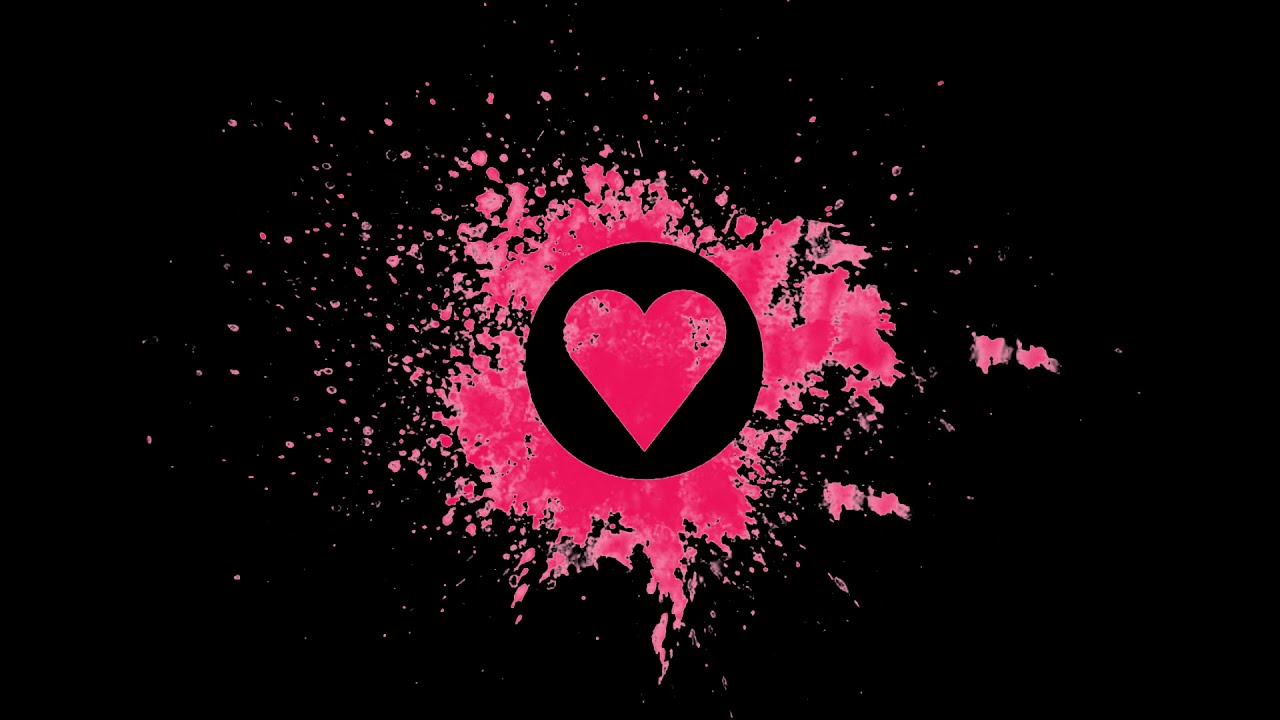The artwork is a digital piece set against a black rectangular background. It features dynamic splashes of pink paint in various shades, creating an energetic visual effect. At the center of this composition is a black circle with a heart-shaped cutout through which the splattering of dark and light pink tones remains visible. These pink splatters radiate outward from the black circle, gradually reducing in size and intensity, giving a sense of movement and vibrancy. The heart within the black circle is also painted in shades of pink, with varying densities of paint, allowing glimpses of the black background through lighter splatter areas. The combination of pink tones and the heart cutout framed by the black circle against a stark black background creates a striking and cute visual contrast.